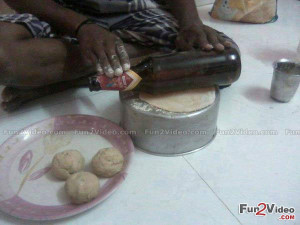The image is a screenshot from a video with the website "fun2videos.com" written in red across the top and "fun2video.com" in red at the bottom right corner. The words "fun" and "video" are in black, outlined in white. The scene depicts a dark-skinned woman with a black band on her right wrist, sitting cross-legged on a white tile floor. She is wearing a black-and-white dress and using a brown bottle with a label around its neck to roll out dough on an upside-down aluminum pot. In the bottom left corner, there is a pink dish with a floral design, holding three balls of dough. An aluminum cup is visible towards the top right of the image, and what appears to be the bottom of a bag is in the top right corner. The woman is meticulously rolling out the dough with the bottle.